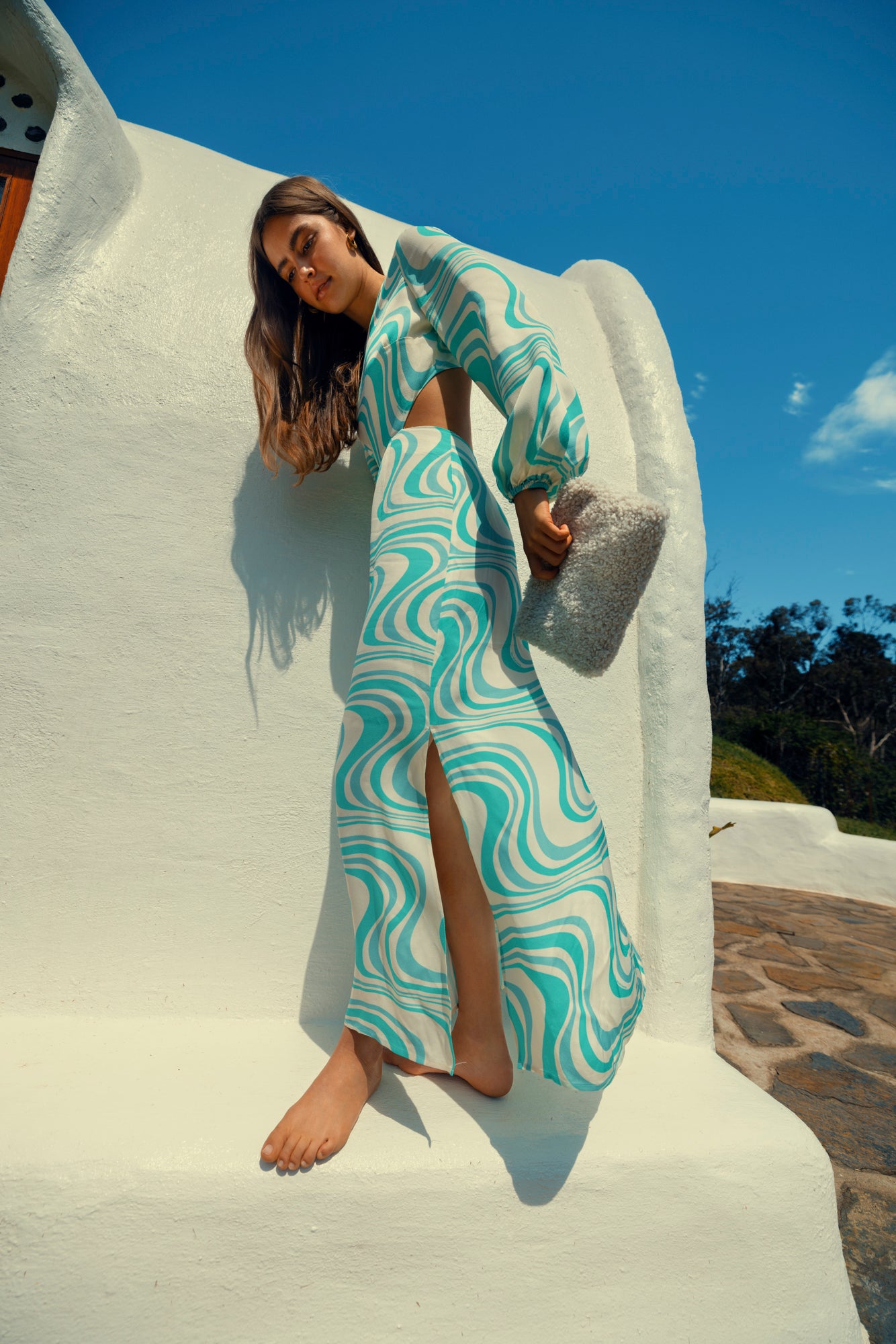In this vivid and bright advertisement shot taken on a clear, sunny afternoon, a young woman in her twenties stands barefoot on a stark white stucco structure, evocative of Mediterranean architecture. The sky is a brilliant blue, almost cloudless, casting sharp shadows behind her. She's wearing a full-length, flowing dress adorned with light pastel turquoise waves and a slit up to her knee on a white background. The dress features puffed, billowing sleeves and a cut-out section in the middle, partially exposing her tanned skin. Her long brown hair, highlighted at the ends, frames her face as she smiles pleasantly. She accessorizes with earrings and a furry clutch in her left hand. The setting includes glimpses of mosaic tiles and a stone pavement or driveway with a touch of vegetation.